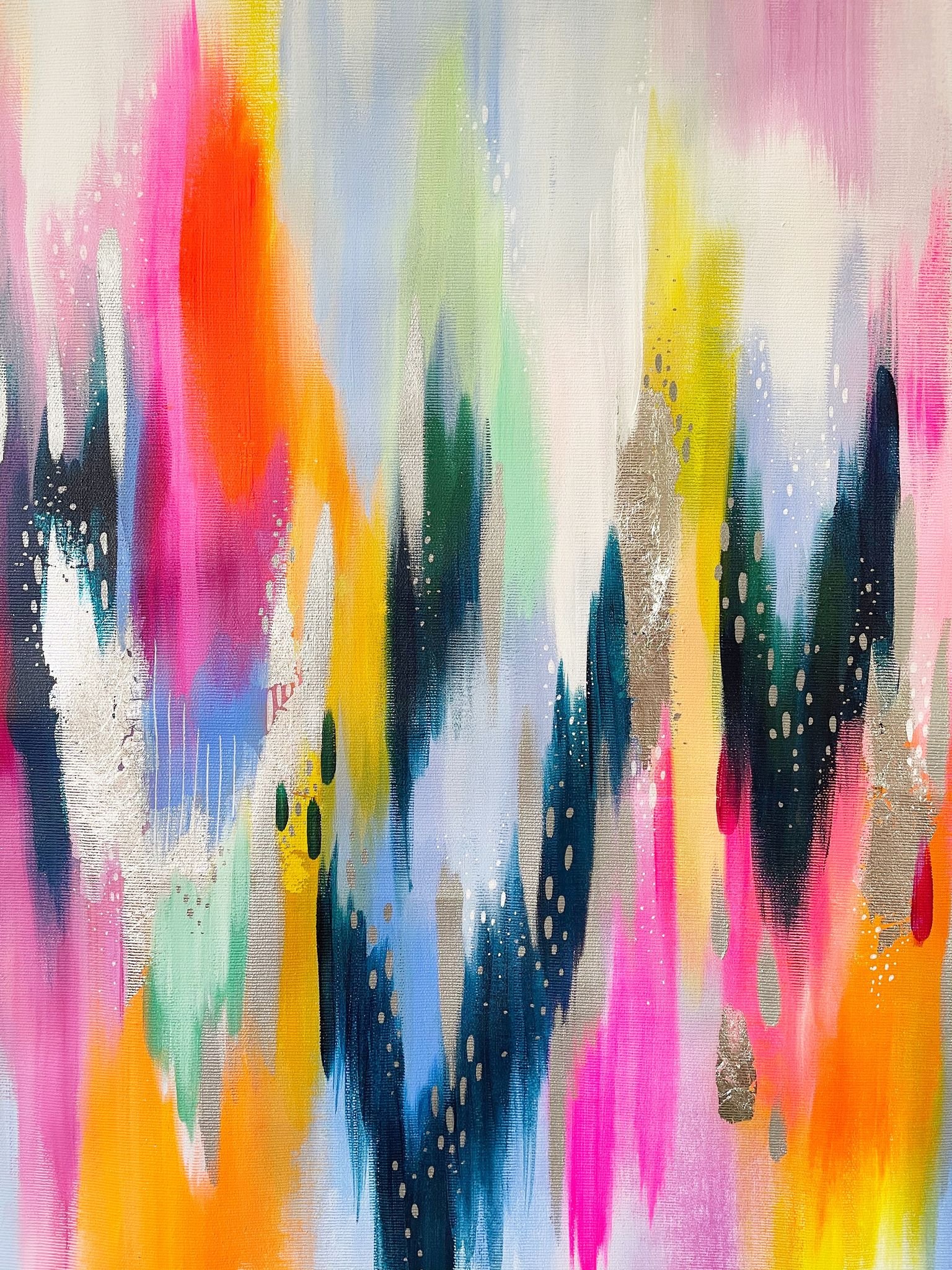The image showcases an abstract oil painting where vibrant colors are smeared vertically from top to bottom, creating a dynamic, dripping effect. In the top right corner, predominant pinkish-orange hues cascade downward, while the bottom right features a blend of orange and yellow descending towards the corner. Centrally, dark blues form a V-shape near the bottom, with a backdrop of lighter blue, interspersed with gray spots. The top left area blends pink, white, and a hint of yellow, continuing the vertical smeared pattern.

The artwork's chaotic yet harmonious color interplay resembles stylized flames, with colors ranging from typical flame shades of orange and red at the top to unusual dark blue, black, and green tones. Noteworthy are the sharp, flame-like shapes, especially in the darker areas, contrasted with interwoven patches of purplish-pink and turquoise.

This oil painting on canvas employs a range of almost every color, with particularly significant regions of red, dark green, and blue. Above the blue sections, splashes of grey and white ink add textural variety. Despite the inherent messiness, the artwork's rich palette and vertical strokes create a vivid and captivating composition that remains unframed.